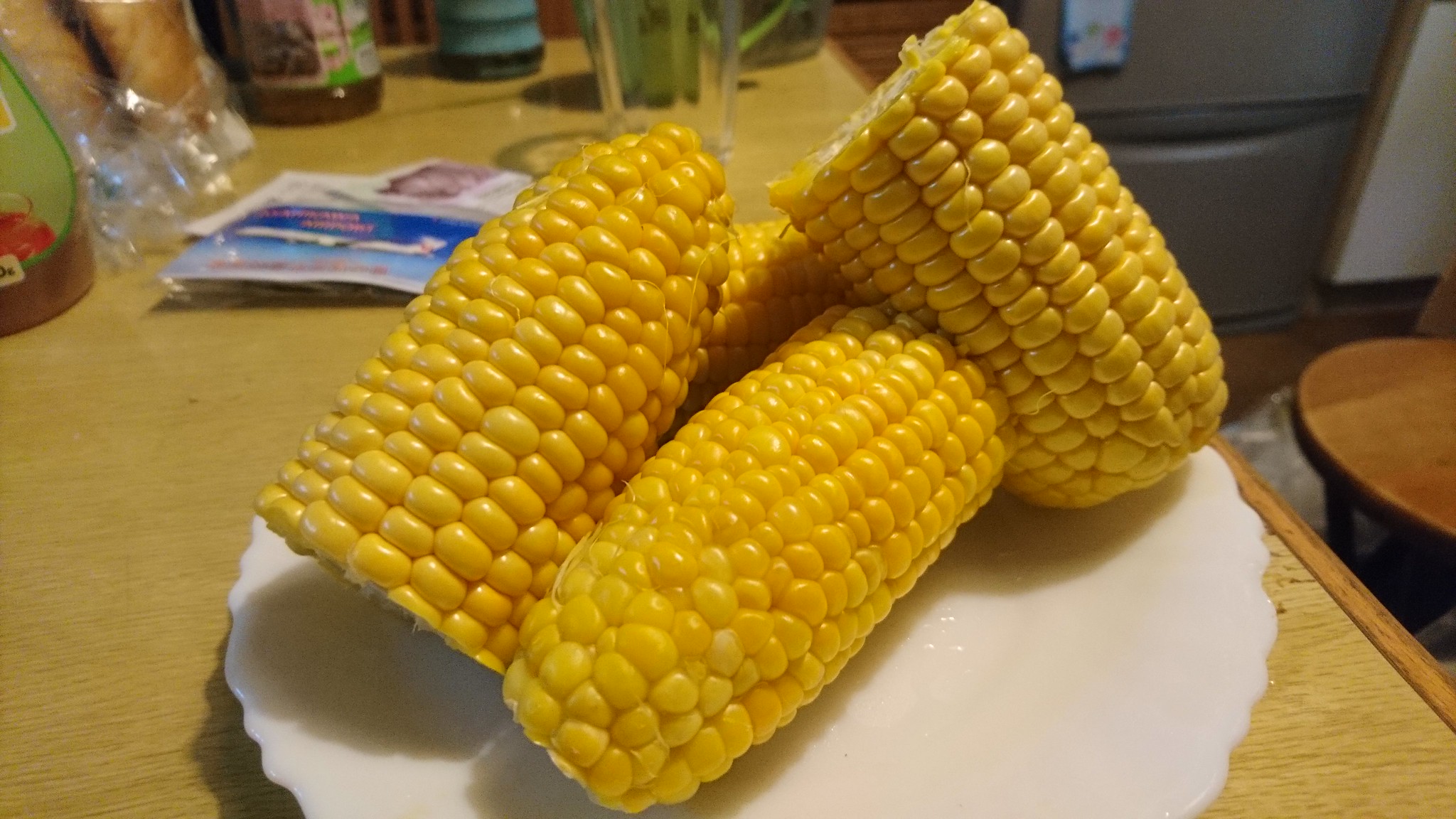In this detailed kitchen scene, a wooden tabletop holds a white, scalloped-edged plate at the center, showcasing four bright yellow corn on the cobs, each cut in half and cleaned, ready for cooking. The table is cluttered with various items: jars with blue, white, and green labels, packets, papers, and an empty glass. In the background, a stainless steel refrigerator is partially visible alongside a brown table and a white wall. A brown wooden floor complements the setup, and a partial round bench hints at a cozy seating area in the kitchen.